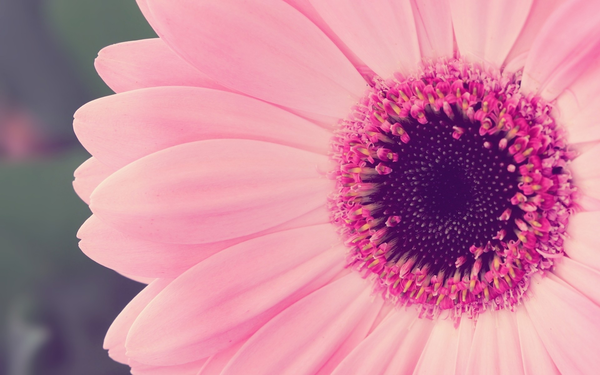This close-up, macro photograph captures the intricate beauty of a pink flower, possibly a daisy. The flower features layers of elliptically shaped petals, which are pale pink with ridges that add to their detailed texture. The centerpiece of the blossom is a dark, possibly brown or purplish core, surrounded by a vibrant ring of hot pink nodules or smaller pigment clusters. These rich details occupy about 75% of the frame, focusing primarily on the flower's detailed and textured center. The background, only faintly visible on the left, is a blurred green, providing little context and emphasizing the flower's delicate structure. The image, enhanced perhaps with a filter, may originally depict a white flower, adding to its visual allure and simplicity.